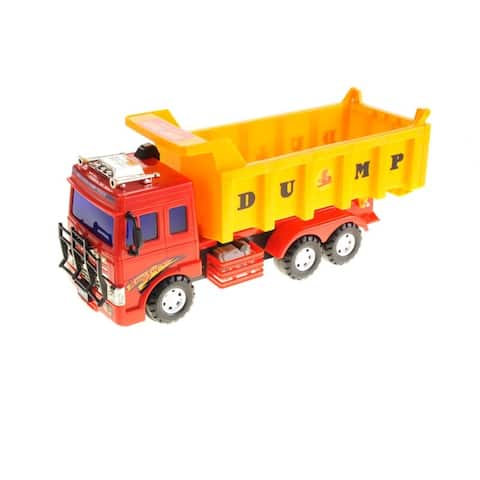This image features a detailed toy dump truck set against a pure white background, highlighting just the truck. The main body of the truck is painted vibrant red, while the container or dumping attachment at the back is bright yellow. Large, black letters spelling "D-U-M-P" are prominently displayed on the side of the container. The truck boasts tinted, dark blue windows, including both a front windshield and side windows which obscure the interior view. 

On the front of the truck, there's a black bumper, and a black grill located where the radiator would be. Additionally, the truck is equipped with black spoke tires featuring white hubcaps. The rear of the truck shows two sets of wheels, suggesting a total of six tires. 

A silver fixture, which appears to be a suitcase rack or possibly related to the truck's cabin horns, sits atop the vehicle, adjacent to the black ear horns. Black side mirrors extend from where the driver’s seat would be. The entire toy truck appears to be made of plastic, and is designed with a meticulous eye for detail, right down to the small black mirrors and the functionality of the dumping container.